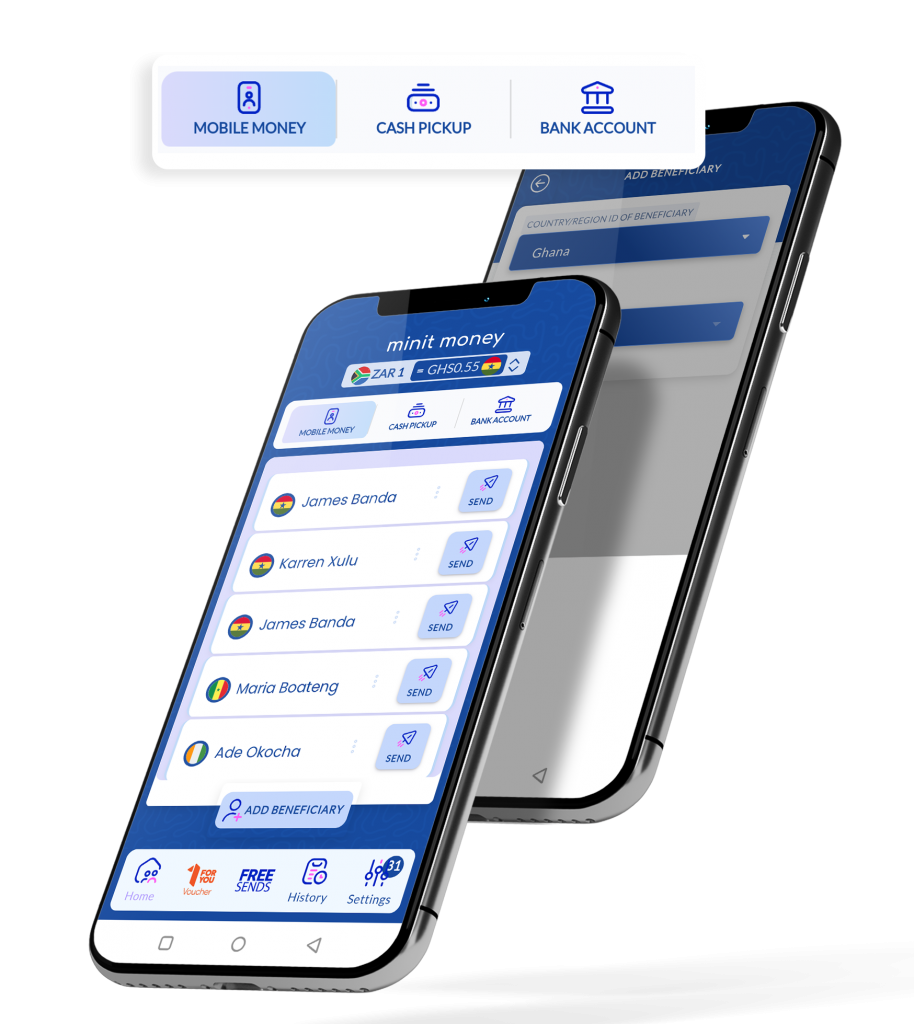The image features two smartphones, both slightly angled to the right. The top phone's screen displays a section labeled "MINUTE MONEY" and has a visible bar of information beneath it. Below this, the phone shows three options: "MOBILE MONEY" (highlighted in blue), "CASH PICKUP," and "BANK ACCOUNT," all in uppercase. The highlighted "MOBILE MONEY" tab contains a list of names, each accompanied by a 'Send' button on the right. At the bottom of this list, there is an option to "Add a Beneficiary." 

The second phone underneath appears grayed out and less visible but contains text that reads: "Country/Region of Beneficiary," specifically mentioning "Ghana," indicating the user can categorize beneficiaries by country. 

At the very top of the image, there's a white rectangular banner encompassing three sections: the first shaded in blue labeled "MOBILE MONEY," and the next two in white labeled "CASH PICKUP" and "BANK ACCOUNT," all in capital letters.

The bottom of the screen on the first phone features three prominent icons, likely for navigation or additional settings. The entire setup seems designed to manage and send mobile money, with clear options and functionalities for sending funds to different beneficiaries or regions.